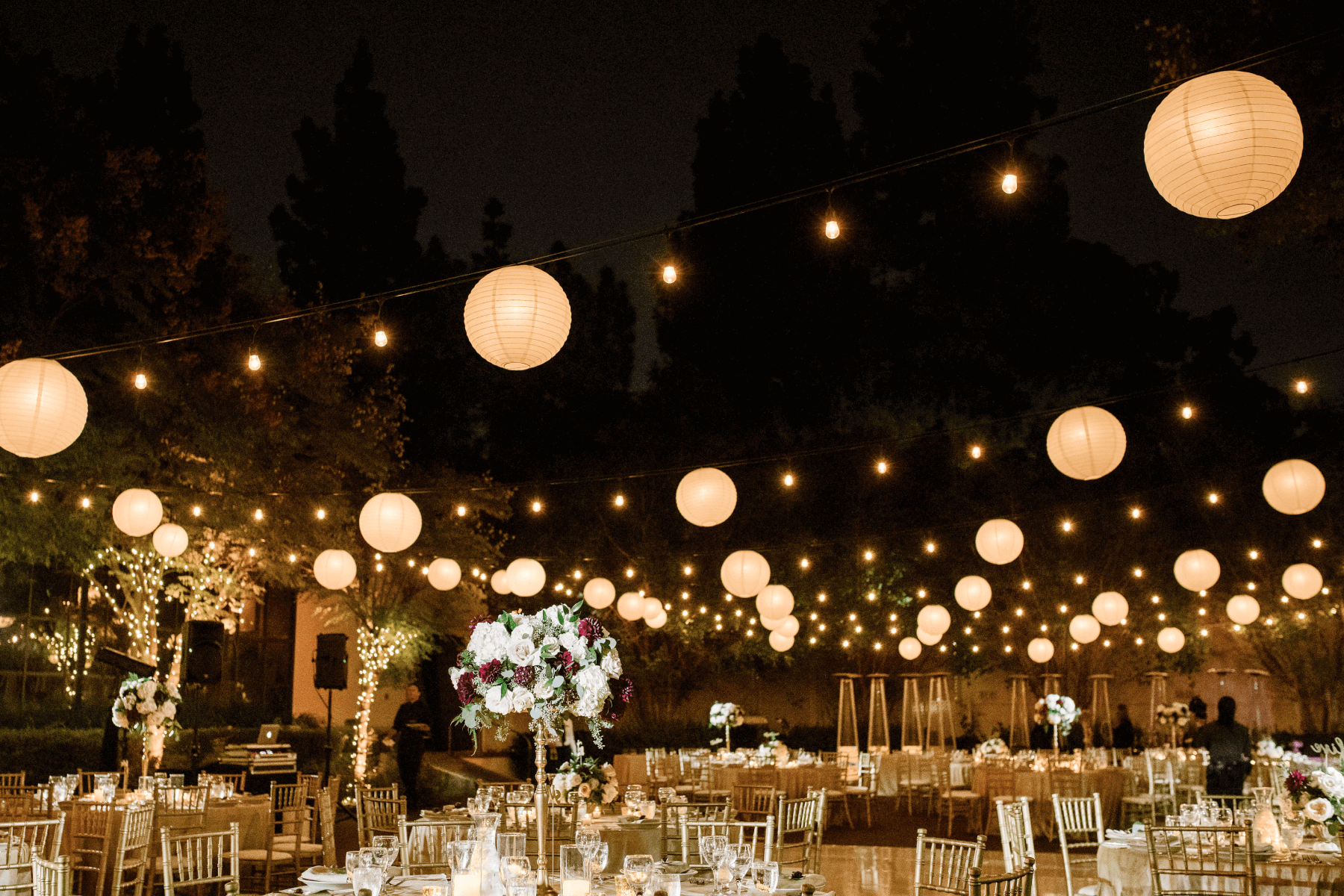The photograph captures a picturesque wedding reception set in an outdoor, open-air venue. The scene is adorned with an array of hanging lights, including Chinese-style lanterns, garden lights, and large globe string lights that span across the venue. Some of the lights resemble balloon fixtures, adding a whimsical touch. Below the lights, numerous tables are elegantly arranged with wine glasses and intricate centerpieces. The centerpieces feature large bouquets of white and red flowers, green leaves, and baby's breath, all elevated on golden or bronze stands. The tables are surrounded by golden chairs, which could be reflecting the warm lighting. In the background, the night sky is a deep, dark gray, silhouetted by trees wrapped in twinkling lights, reminiscent of Christmas lights. A few people can be seen standing in the distance, contributing to the lively yet intimate atmosphere, while a standing speaker is visible to the left. The overall setting is both enchanting and inviting, making for a memorable evening.